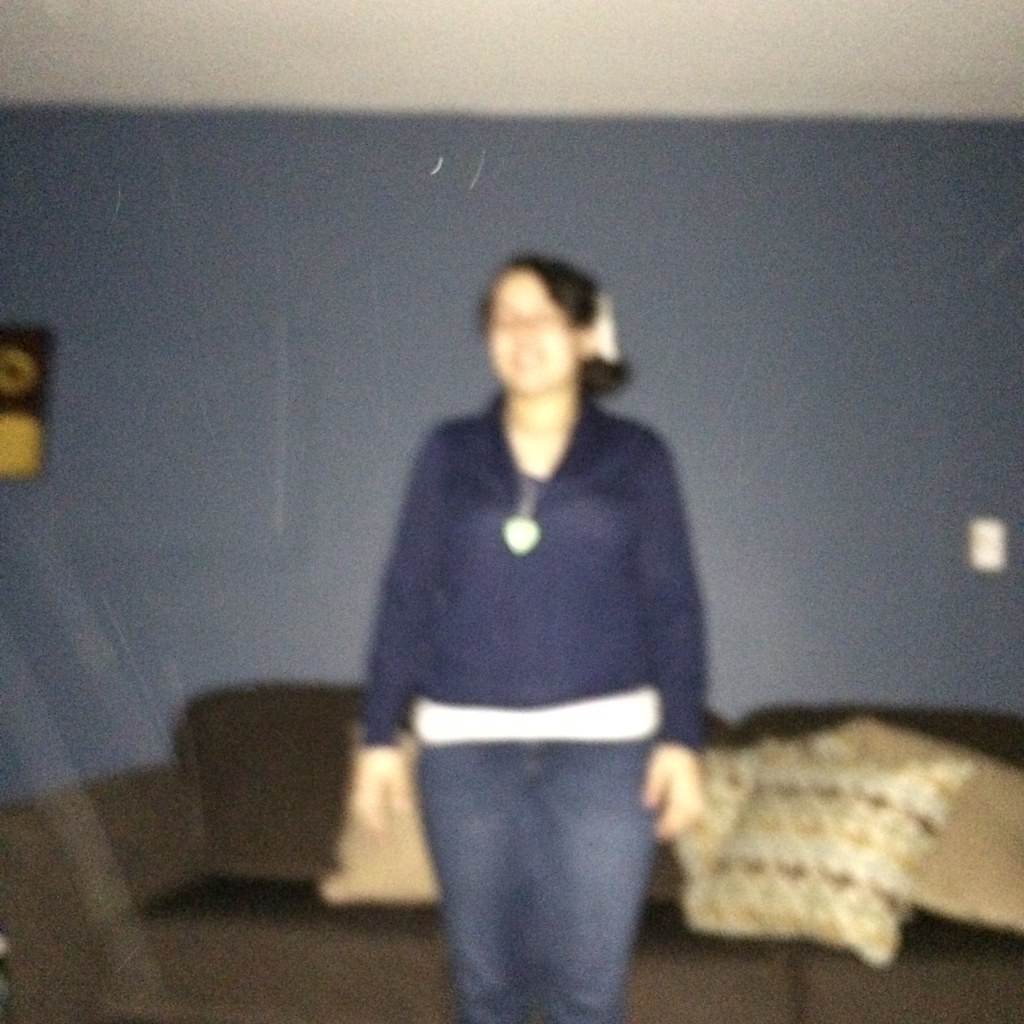A young woman stands in a blurry, out-of-focus image showcasing her casual attire and surroundings. She is wearing a blue jacket over a white shirt, partially visible at her waist, and dark blue jeans. Her short brown hair is styled with a decorative flower clip on one side. The woman has light skin, possibly indicating she is of Caucasian or Asian descent. Behind her, a blue wall and a white ceiling form the background. To the left is a small, square piece of artwork. Below that, a solid brown couch adorned with beige pillows, some featuring intricate designs, completes the scene.